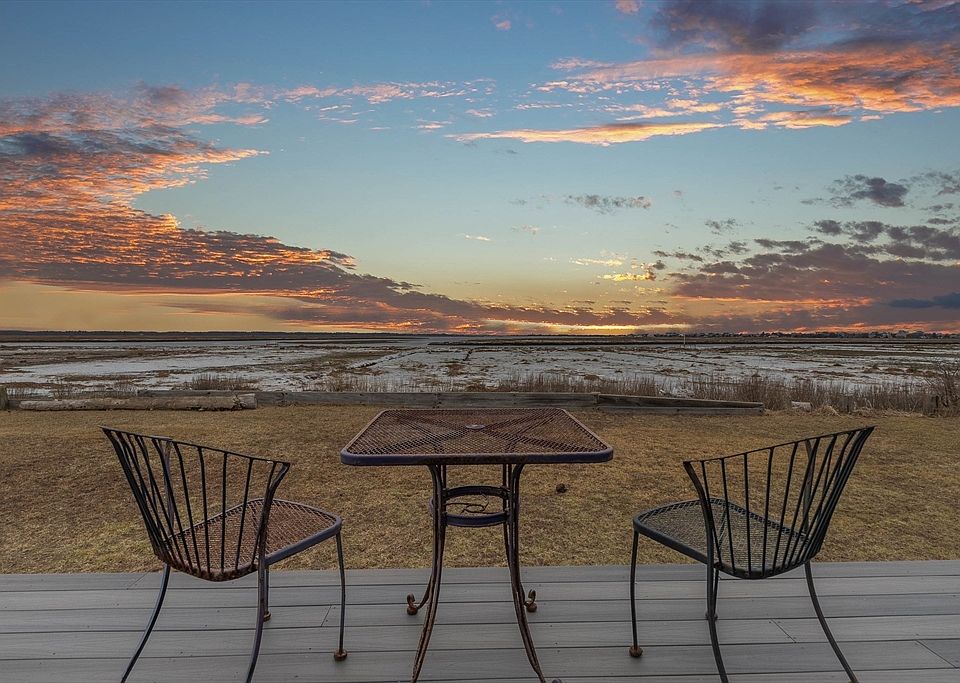This outdoor photograph features a small decked area with new-looking horizontal gray wooden planks, likely someone's porch or patio, devoid of any railing. Central to the image is a small square metal table with a vented top, flanked by two black metal chairs, one to the left and the other to the right, both appearing slightly rusty and without cushions, giving them a rigid and possibly uncomfortable look. Beyond the deck, there's a short green grass yard transitioning into a dirt area. This dirt section appears to have patches of snow and is scattered with weeds and sand. The background showcases a striking sky at sunset, with a blend of clear blue, gray, and orange-pink clouds, creating a dramatic and beautiful natural backdrop. The overall scene exudes a rustic charm, combining elements of man-made practicality and the unrefined beauty of nature.